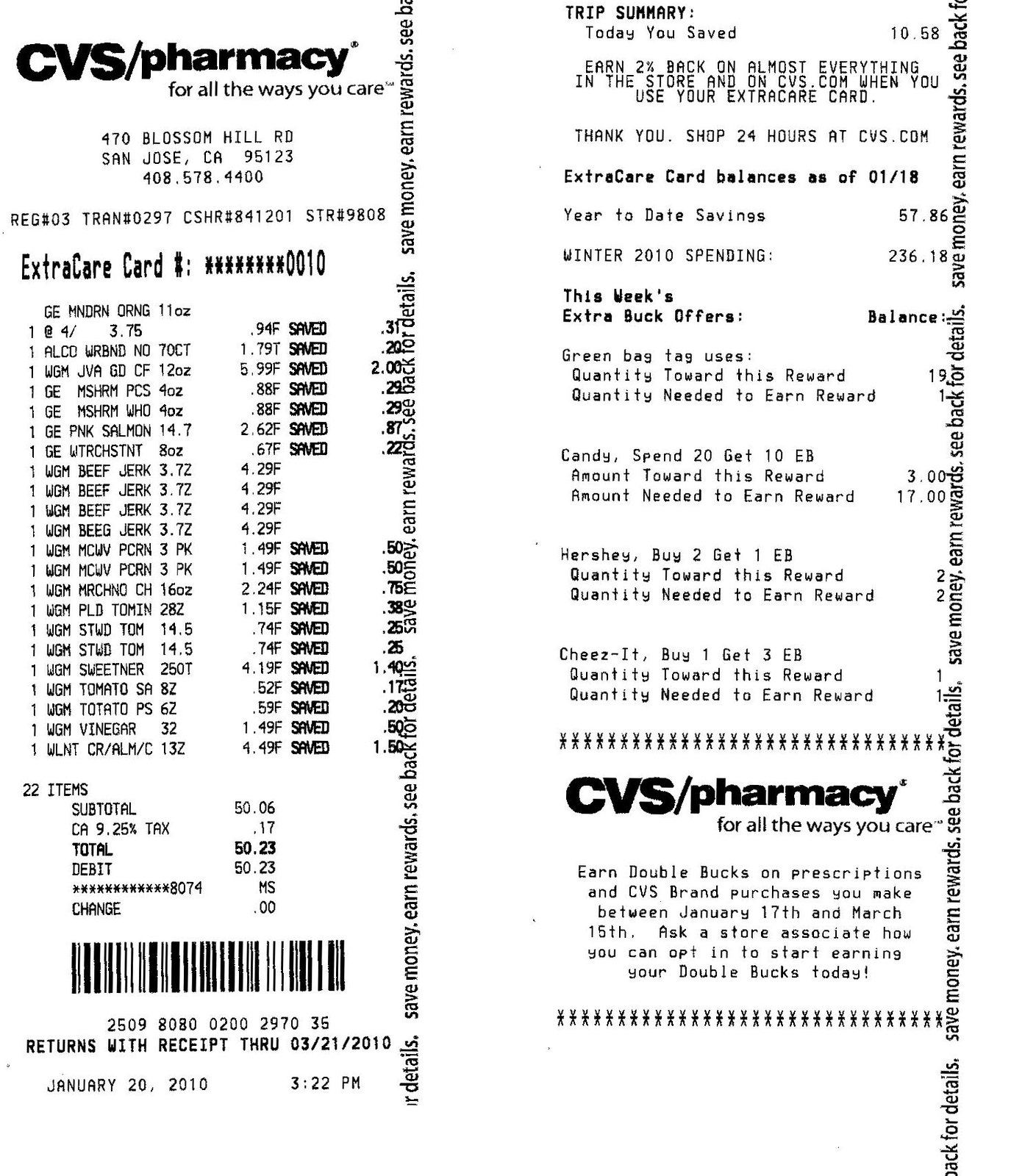A meticulously scanned black-and-white image showcasing a CVS pharmacy receipt split into two halves. The left half prominently displays the CVS store information, specifying the location as 470 Blossom Hill Road in San Jose, California. The ExtraCare card number ends in 0010. Below this, there is a detailed list of the 22 items purchased, with corresponding savings information aligned to the right. The total amount spent is $50.06, with an additional $0.17 tax, bringing the final total to $50.23. Returns are accepted until March 21, 2010.

The right half of the receipt contains a trip summary and additional text. It informs the customer of the savings accrued during the visit, totaling $10.58, followed by a message thanking them for shopping. Further down, the receipt details the ExtraCare card balances and ExtraBuck offers, such as the 'Spend $20, get $10 ExtraBucks' deal, and promotions like 'buy one, get three ExtraBucks' for Cheez-Its. Also, there is information about the CVS Pharmacy survey and the opportunity to earn double bucks on prescription purchases.